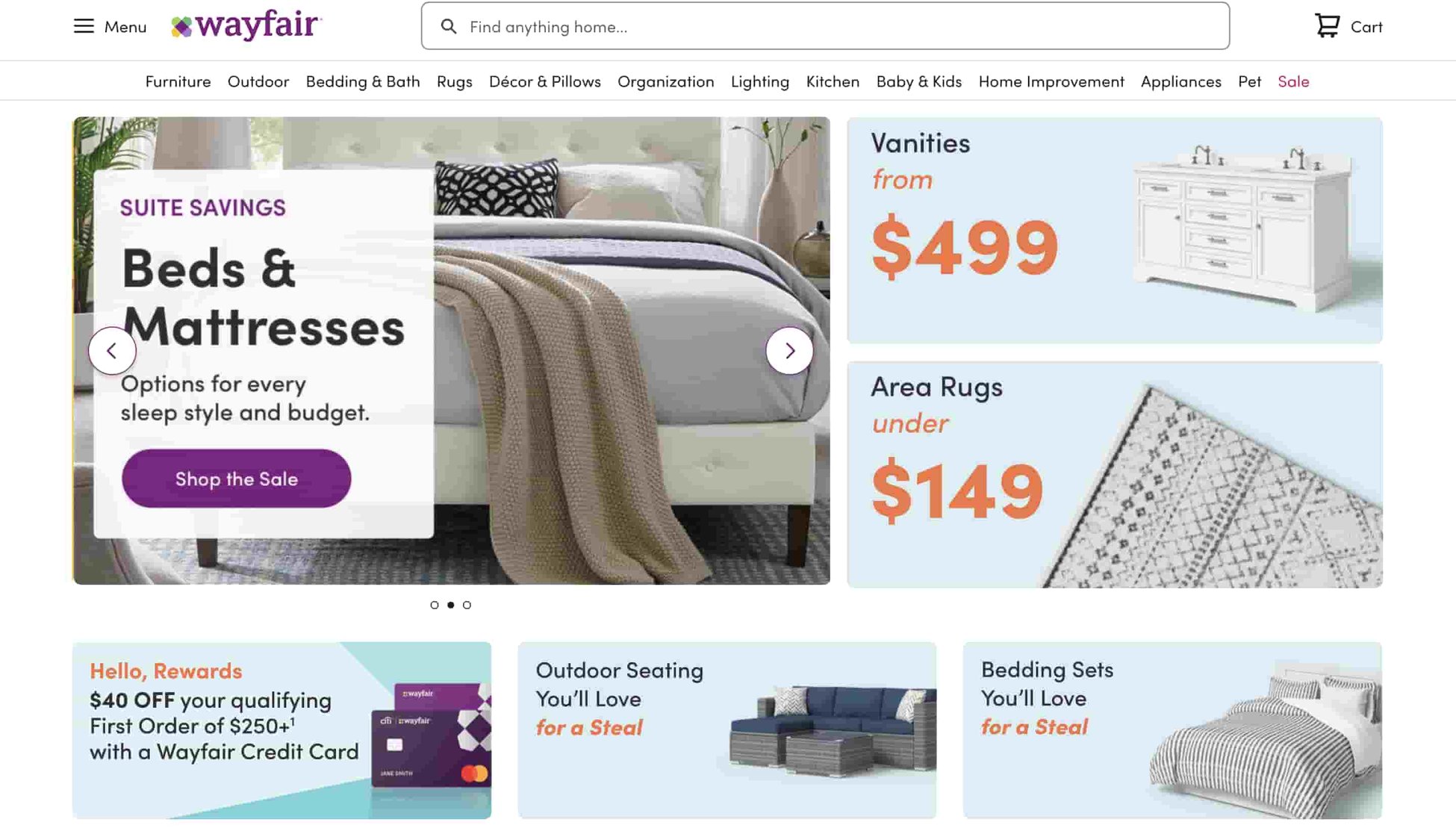This image showcases an online shopping page from Wayfair. In the top left corner, there is the Wayfair logo and a navigation menu categorized into several departments: Furniture, Outdoor, Bedding & Bath, Rugs, Decor & Pillows, Organization, Lighting, Kitchen, Baby & Kids, Home Improvement, Appliances, and Pets. 

On the main section of the page, numerous promotions and deals are highlighted, including:
- Suite Savings: Special discounts on various furniture suites.
- Beds and Mattresses: A range of options tailored to different sleep styles and budgets.
- Vanities starting at $499.
- Area rugs available for under $159.
- Hello Rewards: An offer of $40 off your first qualifying order of $250 or more with a Wayfair credit card.
- Outdoor seating that customers will adore.
- Bedding sets that are both stylish and affordable.

The layout is user-friendly, designed to entice and inform customers of the various deals available.